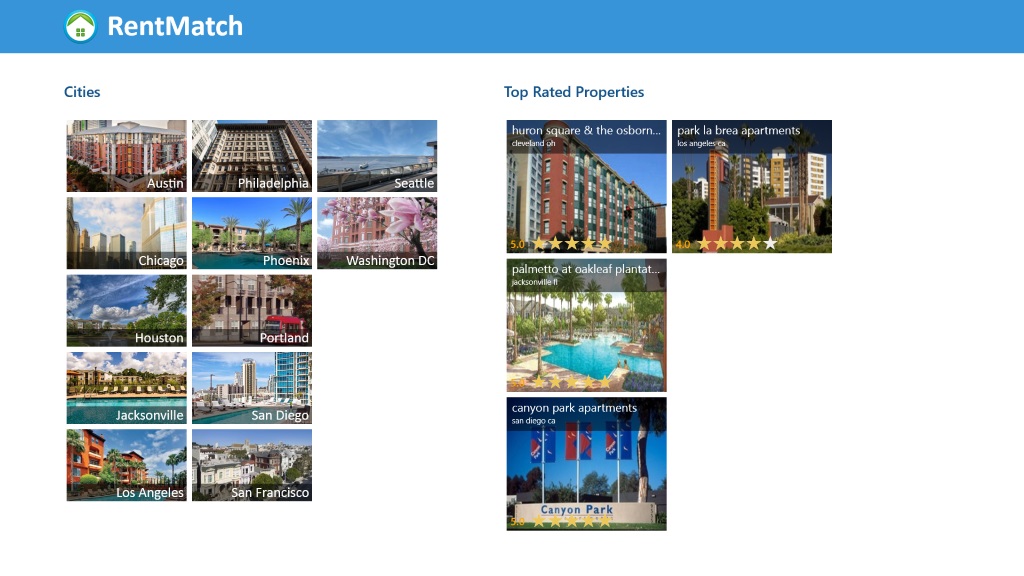This image features a screenshot of the RentMatch website. At the top, there is a blue header with the website's name, "RentMatch," displayed in white text in the upper left corner. Adjacent to the name is a circular logo depicting a house with windows.

Beneath the header, on a white background, the word "Cities" is prominently displayed in blue text in the upper left corner. The main section showcases several city thumbnails with corresponding images:

- In the upper left corner, a thumbnail labeled "Austin" is present.
- To the right, a thumbnail for "Philadelphia" shows a high-rise gray building.
- Continuing to the right, a thumbnail for "Seattle" displays a dock with water.

In the next row:

- "Chicago" is depicted with a view of its iconic skyline.
- "Phoenix" follows.
- "Washington D.C." features a cherry blossom tree.

Following that:

- "Houston" and "Portland" are shown side by side.
- "Jacksonville" features an image of a pool.
- To the right, "San Diego" is represented with a skyline.

Further down:

- "Los Angeles" and "San Francisco" conclude the array of city thumbnails.